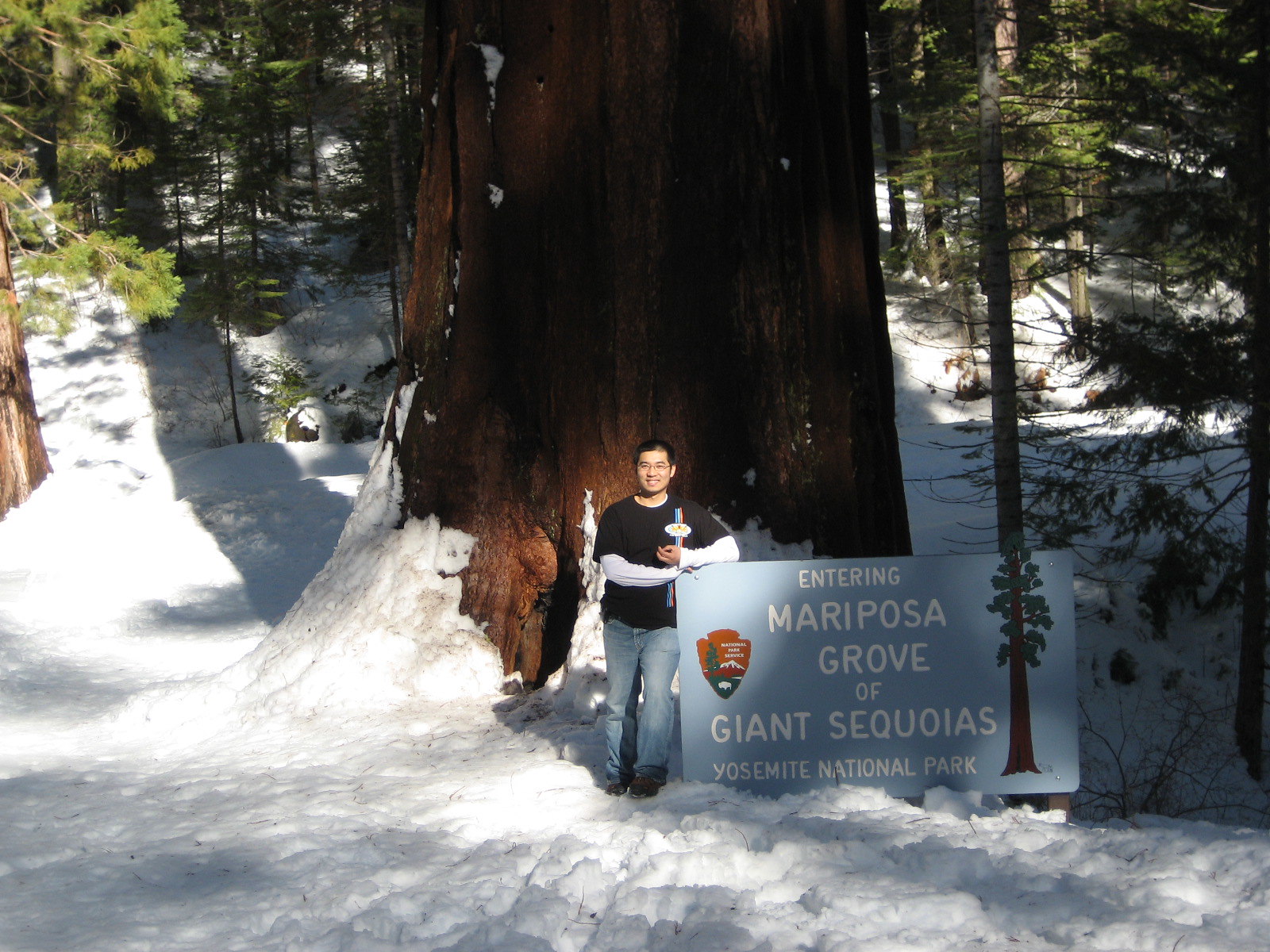This is a color photograph taken on a sunny winter day at Yosemite National Park. The image features an Asian gentleman with short black hair, smiling as he leans against a large wooden sign bearing the National Park Service logo. The sign reads "Entering Mariposa Grove of Giant Sequoias, Yosemite National Park." Behind him stands a majestic giant sequoia tree, part of a forest blanketed in at least a foot of snow. The man is dressed in a black and white long-sleeve shirt, light blue denim jeans, and brown boots, enjoying the bright sunlight that reflects off the snowy ground.